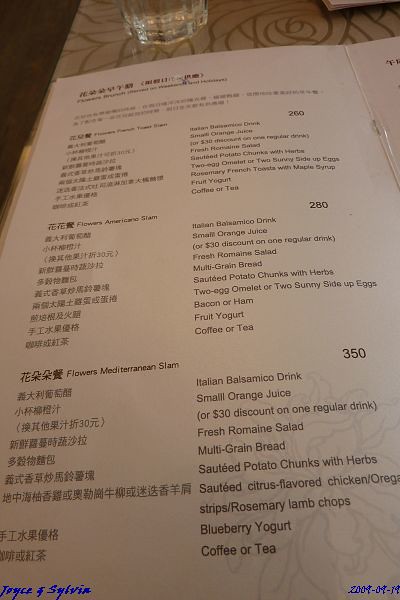"Photograph of a bilingual menu, featuring both English and an East Asian language, possibly Japanese or Chinese. The menu, positioned on a table with a glass partially covering it, lists various breakfast options. 

Visible items on the menu include:
- Small orange juice
- Fresh romaine salad
- Multigrain bread
- Sautéed potato chunks with herbs
- Two egg omelet or two sunny side up eggs
- Bacon or ham
- Fruit yogurt or coffee or tea

The menu features offerings titled 'Flowers Mediterranean Slam' and lists three variations of set meals, each repeated three times on the left-hand side:
1. A set meal priced at 260 (currency unclear)
2. 'Flowers American Slam' priced at 280
3. 'Flowers Mediterranean Slam' priced at 350

Additional details for the first set meal include rosemary French toast with maple syrup, and the third set meal offers sautéed citrus-flavored chicken strips and rosemary lamb chops. Notable text includes blue writing in the bottom left corner that says 'Joyce and Sylvan,' and the menu is timestamped 2009-09-19 in the bottom right corner. The right-hand side of the menu is not visible in the photograph."